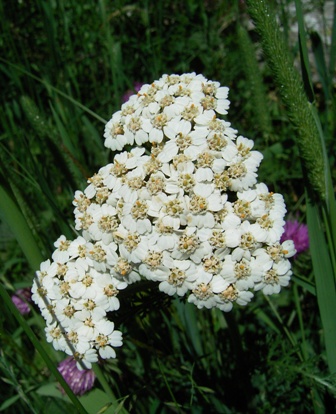In this vibrant outdoor photograph, a cluster of white flowers with yellow and brown centers takes center stage. Nestled among them are a few pink or purple flowers, particularly noticeable in the bottom left corner, middle left, and bottom right of the floral grouping. Tall, thick grass surrounds the cluster, with a noticeable pollen grain on the top right corner of one grass blade. The background is a lush green, dotted with additional pink or purple flowers on the right, top, and left corners. The top right corner hints at rocky terrain or parts of a mountain, adding depth to the scene.